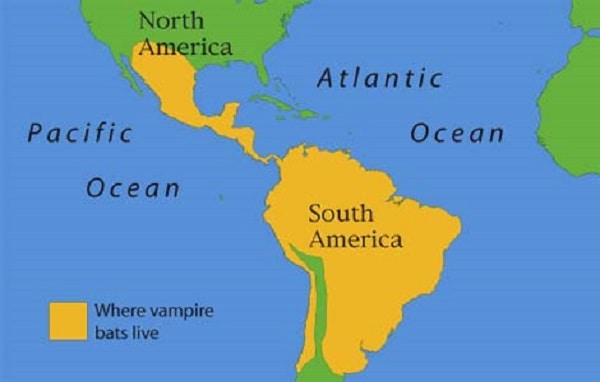The image depicts a simplified map highlighting the geographic distribution of vampire bats. It features a blue background representing the water bodies, with North and South America prominently displayed. North America is predominantly green, with the southwestern region extending through Mexico and Central America highlighted in yellow. South America is primarily yellow, except for a narrow green strip running along the Andes Mountains. Labeled oceans include the Pacific Ocean to the left and the Atlantic Ocean to the right. Partial depictions of Africa and Europe, shown in solid green, are visible to the right of the map, although they are cut off. A key in the bottom left corner, marked with a yellow square, specifies that the yellow regions indicate areas where vampire bats live. This map appears simplistic and might be designed for educational purposes, possibly in a child's textbook.